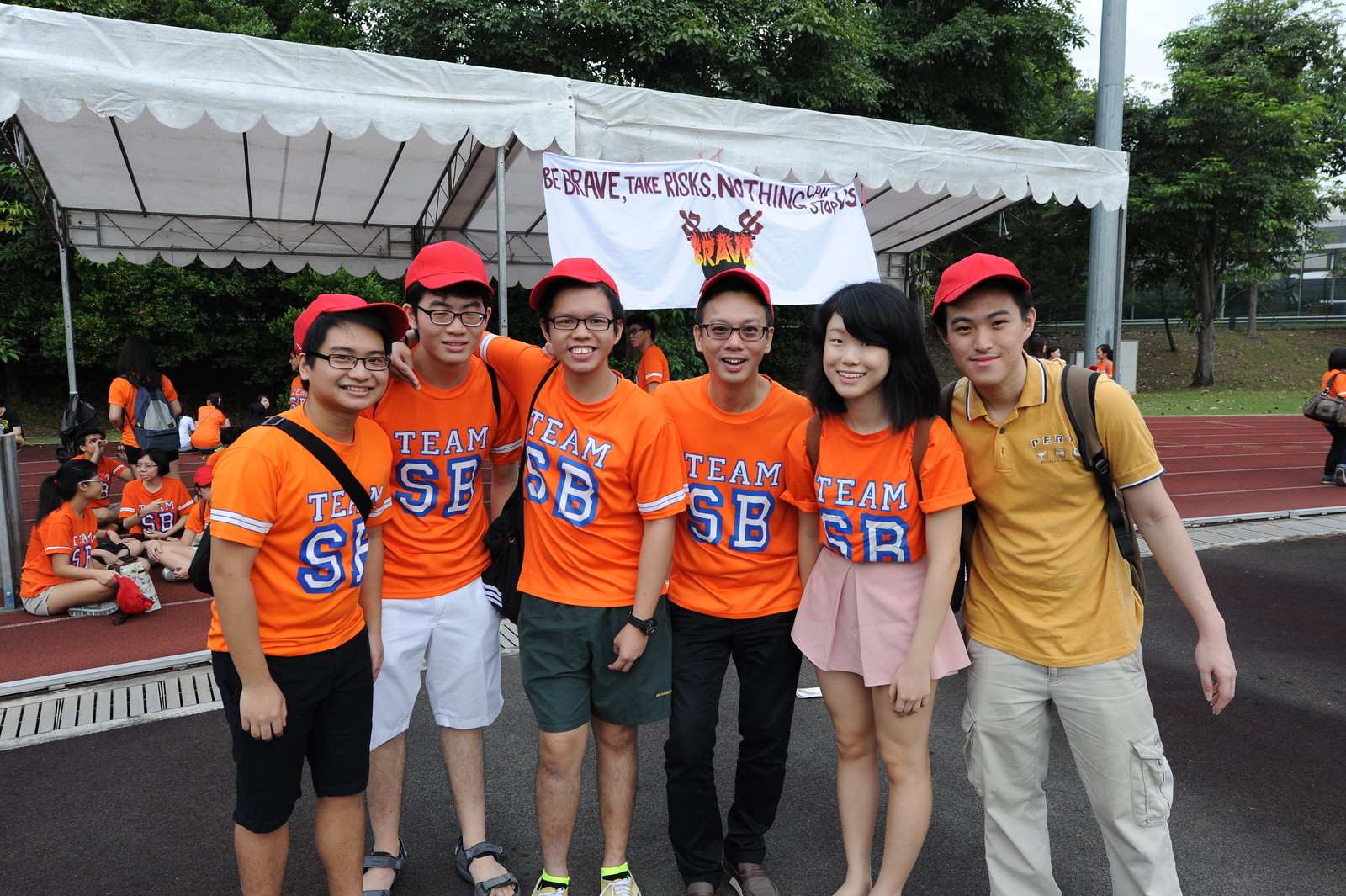This photograph features a group of six young individuals of apparent Asian descent, standing proudly in front of a white tent amid a backdrop of trees and a track. A visible banner on the tent reads, "Be Brave, Take Risks, Nothing…," with the remaining words obscured. Below the banner, the word "Brave" is highlighted in black and orange. The team consists of five boys and one girl, with five members wearing bright orange short-sleeve jerseys emblazoned with "Team SB" and corresponding red hats. Their outfit specifics include black, white, and hunter green shorts, with one boy in the center donning black pants. The girl stands out in a pleated pink skirt and no cap. Positioned to the far right, the sixth individual sports a yellow polo shirt and khaki cargo pants, also wearing a red hat. In the lower left background, additional team members dressed in orange shirts are seated under the tent, suggesting a group larger than the initially visible six. The setting seems to be related to an athletic event, indicated by the track and other people seen in the background. All members are smiling, showcasing camaraderie and team spirit.